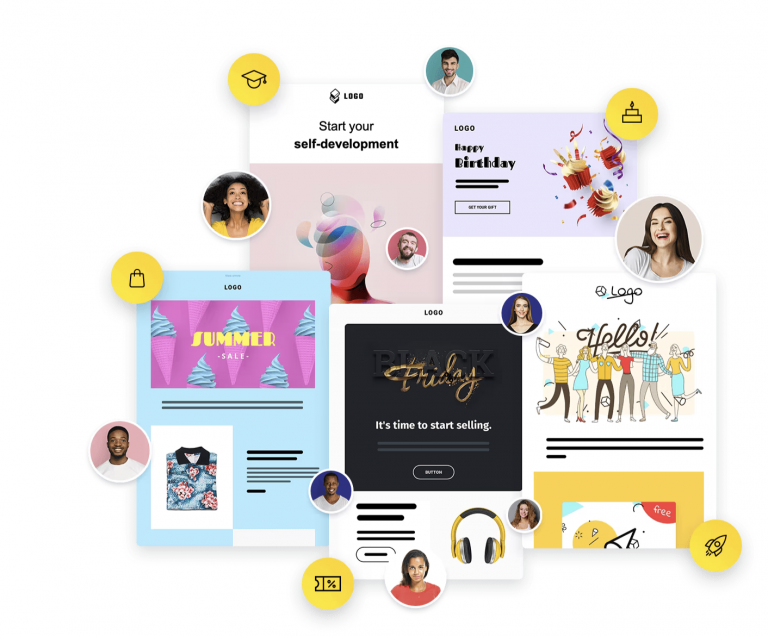In this screenshot, which appears to be an advertisement or a social media post, the composition is filled with vibrant and colorful elements. 

At the top, there is a profile image of a young man with a dark beard, mustache, and dark hair, enclosed in a circular frame. 

On the left side, a white and pink box displays the text "Logo. Start your self-development." Inside the pink box, there are images of two individuals: a man who looks to be in his 40s with a brown beard and mustache, and a young woman with brown curly hair, wearing a yellow shirt, similarly enclosed in circular frames.

Below the female's circle, there is a light blue box that reads "Logo. Summer Sale" and features a graphic of blue ice cream cones on pink backgrounds.

In the center of the screenshot, against a black backdrop, bold text reads "Black Friday. It's time to start selling."

In the upper right corner, a lavender box showcases an image of cupcakes. The upper left corner of this lavender box is labeled with the text "Logo. Happy Birthday!"

The overall design is a mix of promotional messages, vibrant graphics, and diverse subjects, making for an eye-catching and detailed visual presentation.